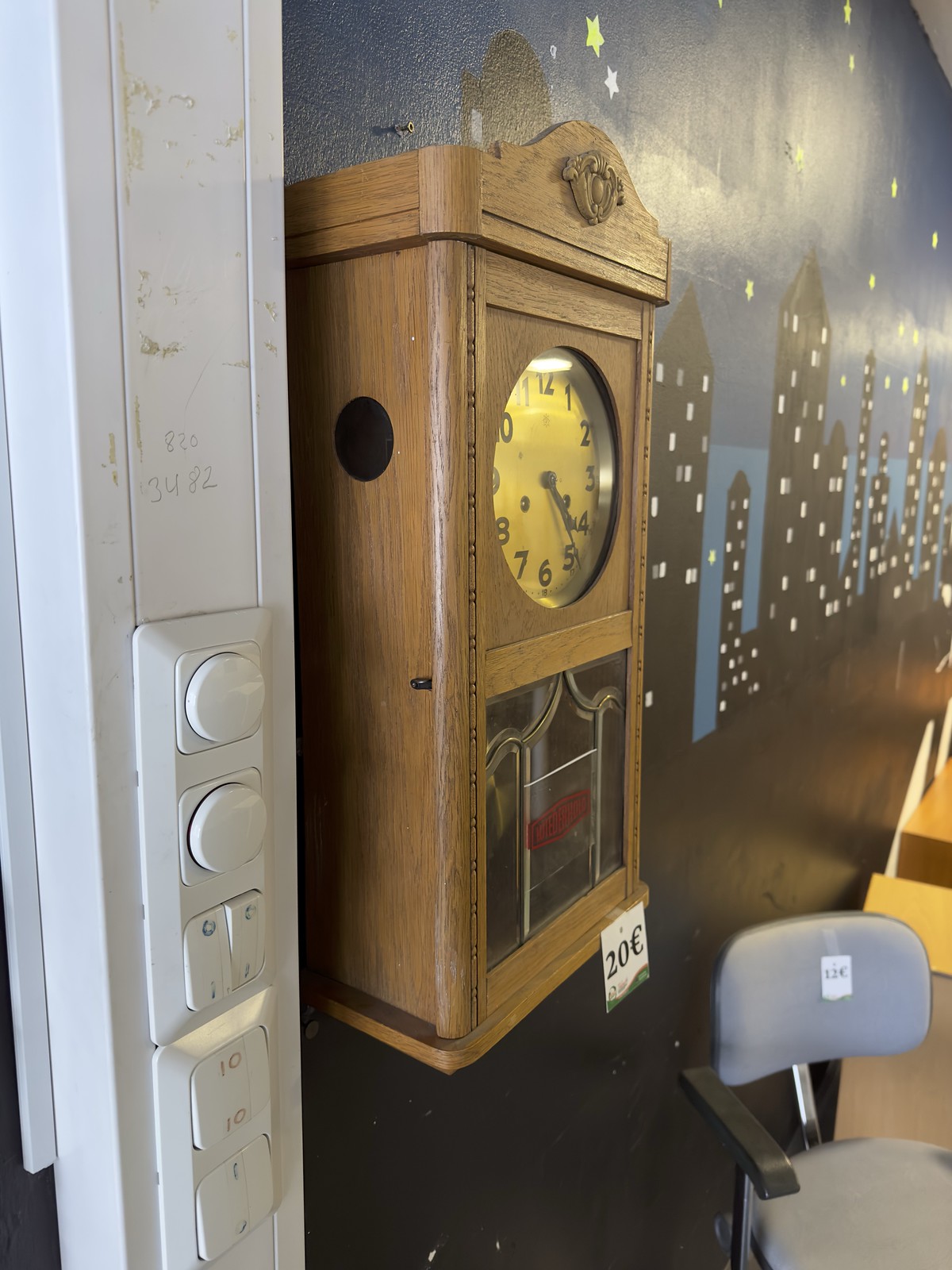The image features a detailed side view of a tall, wooden grandfather clock with a light brown oak finish. The clock has a round, brass-colored face with black numerals and black hour and minute hands, and an open glass section on the lower part where the pendulum is visible. A price tag reading "20 euros" is attached to the lower right of the clock. To the right of the clock, the wall is adorned with a decorative mural depicting a nighttime cityscape. This mural consists of tall, black skyscrapers with triangular tops, illuminated by small white and yellow squares symbolizing lit windows, against a dark blue skyline with stars. Below the clock, a small blue office chair priced at 12 euros sits, featuring a metal pipe connecting the backrest and black armrests. To the left of the clock, a white trim borders a set of various switches and buttons that potentially control the room’s temperature or lighting.